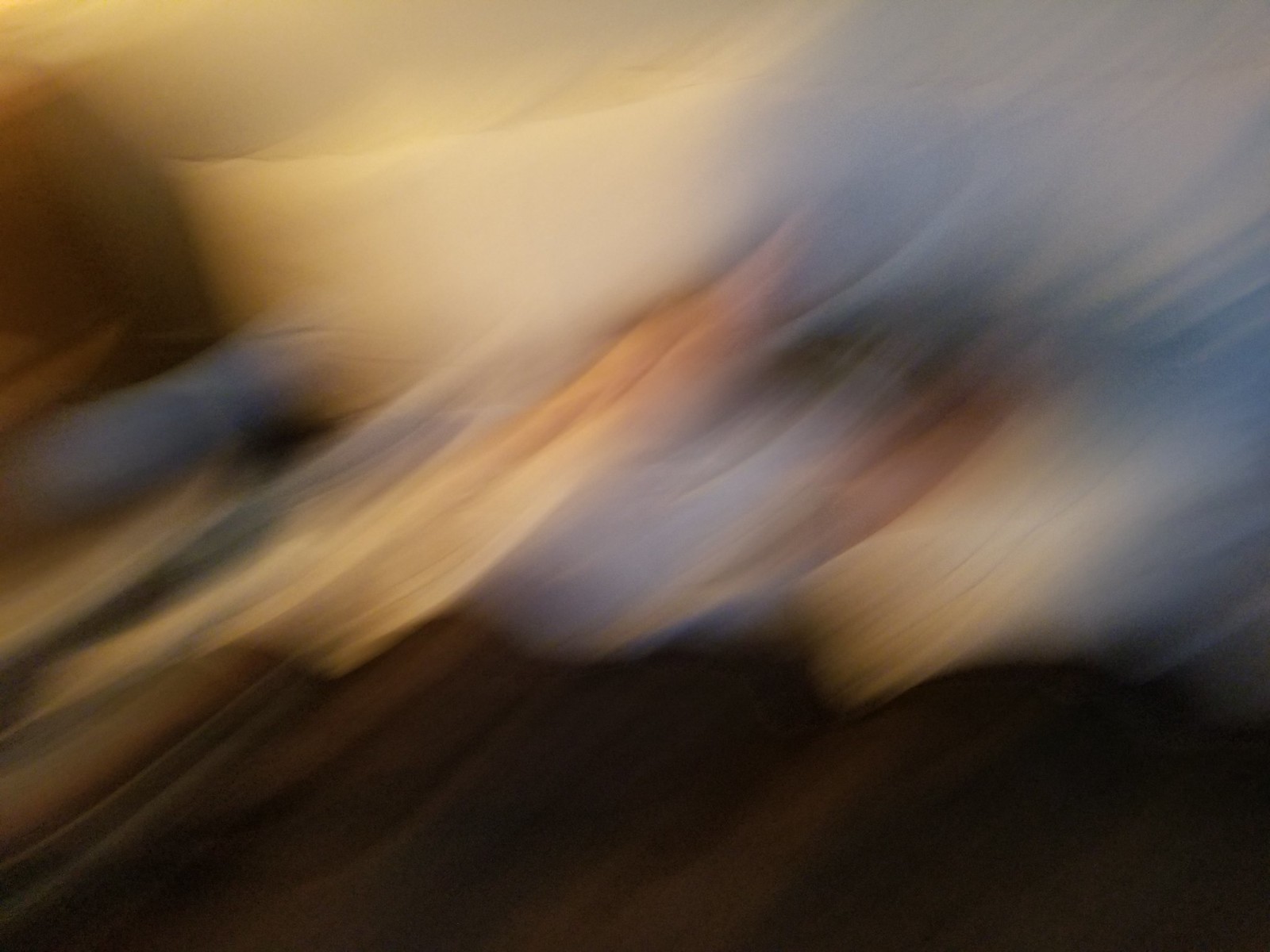The image is extremely blurry, featuring an array of faded and blended colors that suggest either a hurried photograph or an artistic piece meant to convey motion. The upper left corner is predominantly beige, transitioning into a larger section of off-white and light beige, bordered on the left by darker brown with flecks of blue and yellow light. As the blur continues, it forms a tapestry of tan and peach hues, gradually shifting to dark brown toward the bottom. The middle of the image is a mix of blue and yellow, with blue becoming more pronounced at the top right corner, complemented by streaks of peach and beige. There seems to be a diagonal texture to the colors, reminiscent of brush strokes or perhaps fabric folds, with a possible long shadow cast to the right and a general sense of soft, light-bathed surfaces throughout.